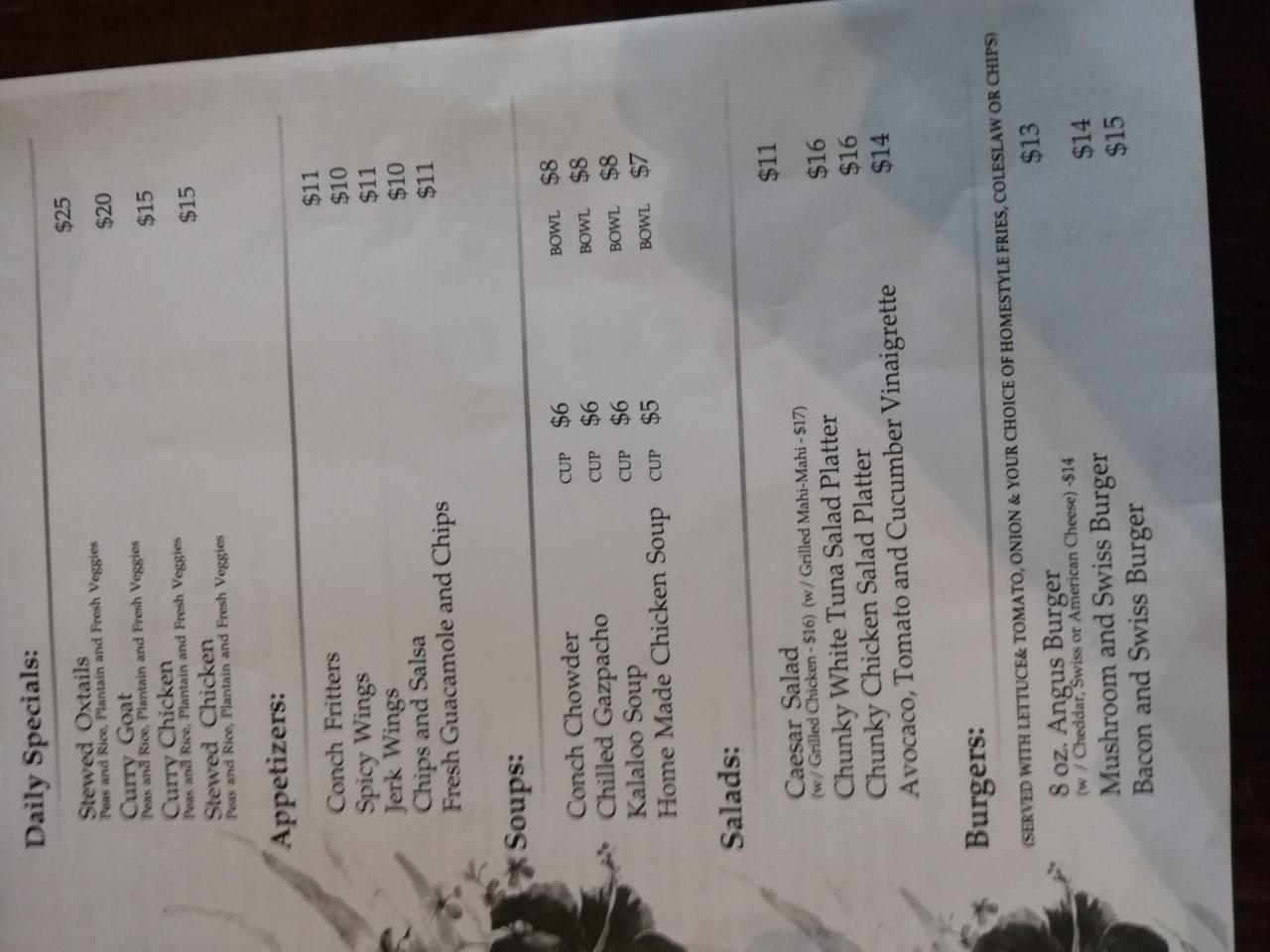This photograph captures a stylish and detailed menu set against a white background in landscape orientation. While the actual menu is designed in portrait orientation, the image showcases it horizontally. There is noticeable shading or a watermark in the right corner that transitions from black to gray in a reflective pattern. Along the left edge of the menu, a dark, floral pattern adds an elegant decorative touch.

The menu itself features black font on a white backdrop, with bolded headings to delineate different categories. The top section, labeled "Daily Specials," offers four options. Following this, the "Appetizers" category is listed with five choices, each section separated by a border line for clarity. 

Further down, the "Soups" section, highlighted in bold, presents four different options, followed by another bolded and bordered section titled "Salads," which also includes four selections. At the bottom of the menu, the "Burgers" category is bolded and bordered, offering three different choices for diners. This detailed menu layout is visually appealing and easy to navigate, making it simple for customers to find exactly what they're in the mood for.